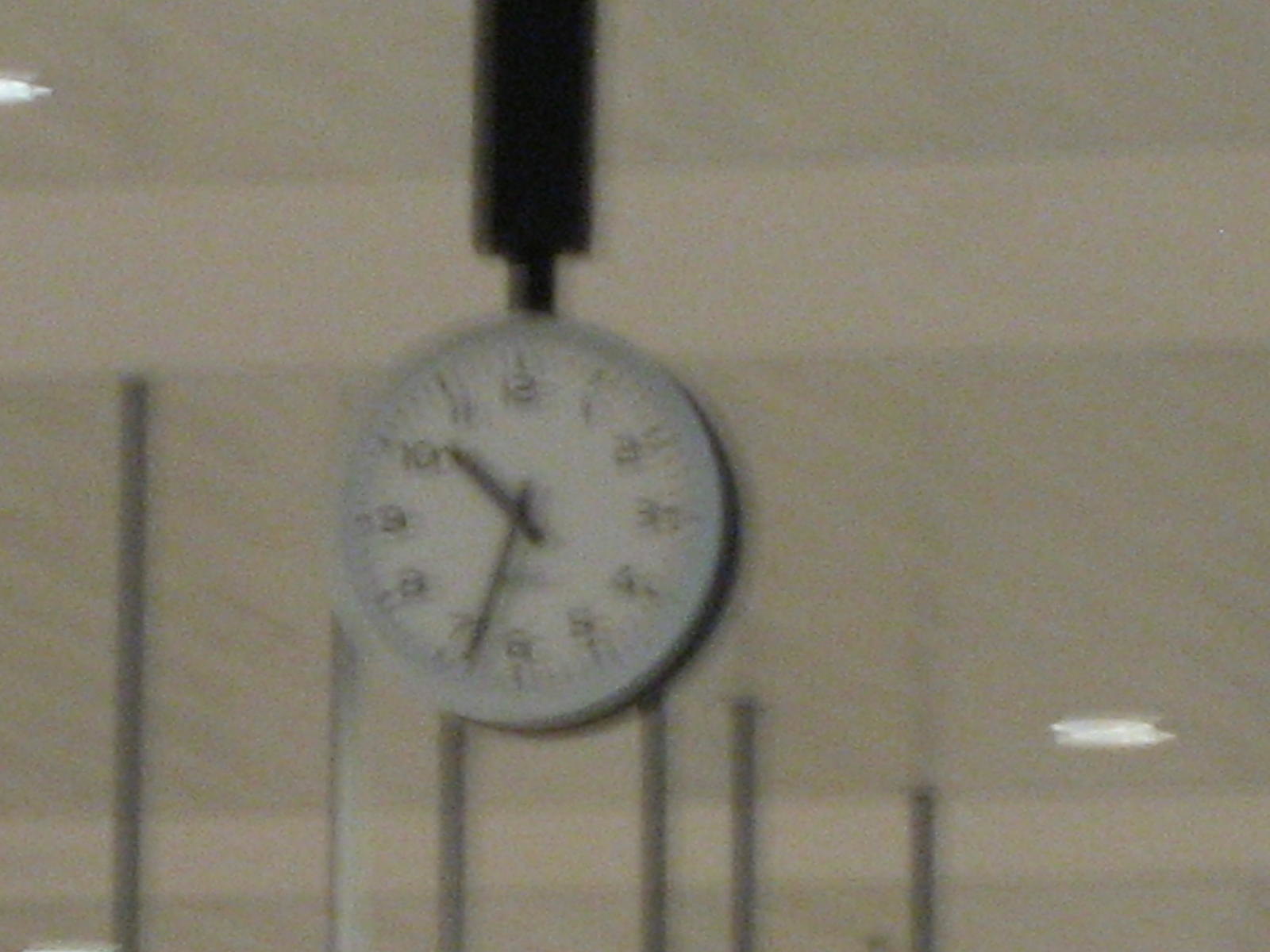A gray concrete building facade with varying levels of textured concrete is showcased in this image. On the right side of the wall, a light fixture is positioned a little over halfway down, while another small light is embedded in the ceiling at the top left corner. A black metal pole descends from the ceiling, supporting a prominent silver clock with a white face. The clock features black numerals and hands, indicating the time as approximately 10:35. The concrete wall is punctuated by several vertical posts and other structural elements, adding to its intricate design.